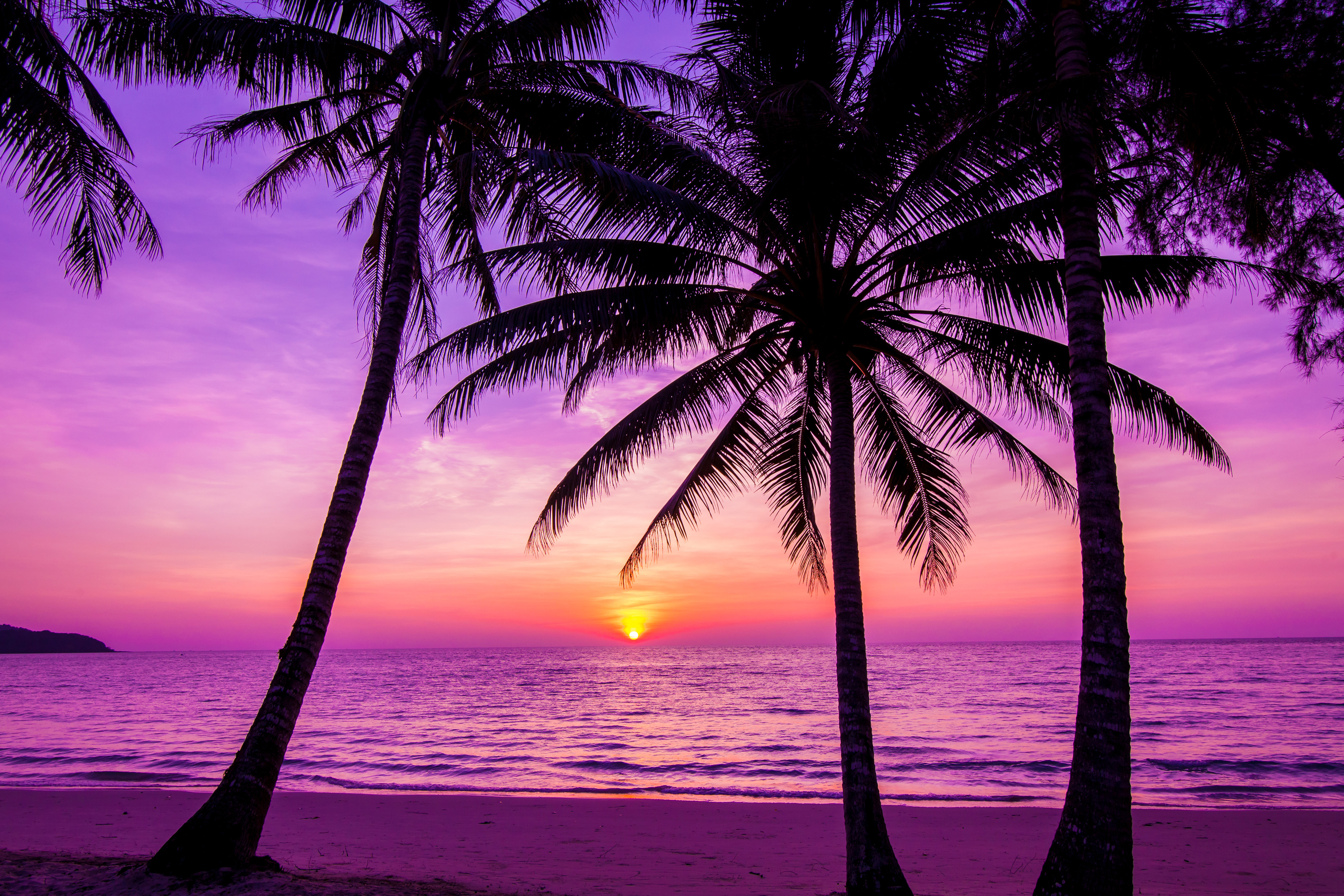This photograph captures a breathtaking beach scene during a sunset, enveloped in a surreal pink and purple hue that suggests the use of a filter effect. Four silhouetted palm trees stretch upward, their dark forms contrasting with the vibrant colors of the sky. The sandy beach, tinted pink, leads to the similarly hued ocean, where the horizon line meets a mesmerizing sky. The sun, a striking orange, sits just above the water, casting rich peach and yellow tones that gradually blend into the purple and magenta clouds. The sky's gradient transitions from deep purples and lavenders to the vibrant sunset colors, creating a harmonious and otherworldly atmosphere. The photograph, rectangular in shape and postcard-pretty, leaves viewers in awe of its stunning and possibly edited color palette that enhances the natural beauty of the scene.